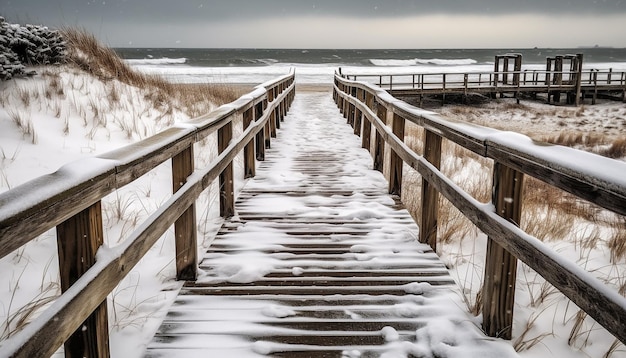The photograph depicts a serene winter scene of a wooden boardwalk extending down to a beach and ocean, enveloped in soft, diffused lighting. The boardwalk's slats are unevenly covered in snow, which also rests lightly on the wooden railings that frame the walkway. Soft focus combined with light grays, medium grays, tans, and whites create a contrasty yet warm glow, suggesting professional photography techniques or post-processing filters were utilized. Flanking the boardwalk are sand dunes partially blanketed in snow, with patches of dune grass and bare, brown stems visible, adding texture and depth to the scene. In the distance, the ocean's dark, wave-capped surface meets a similarly dark gray sky, enhancing the photograph's atmospheric mood. The perspective draws the viewer's eye down the walkway, which continues to a perpendicular path to the right, hinting at further exploration beyond the immediate view.